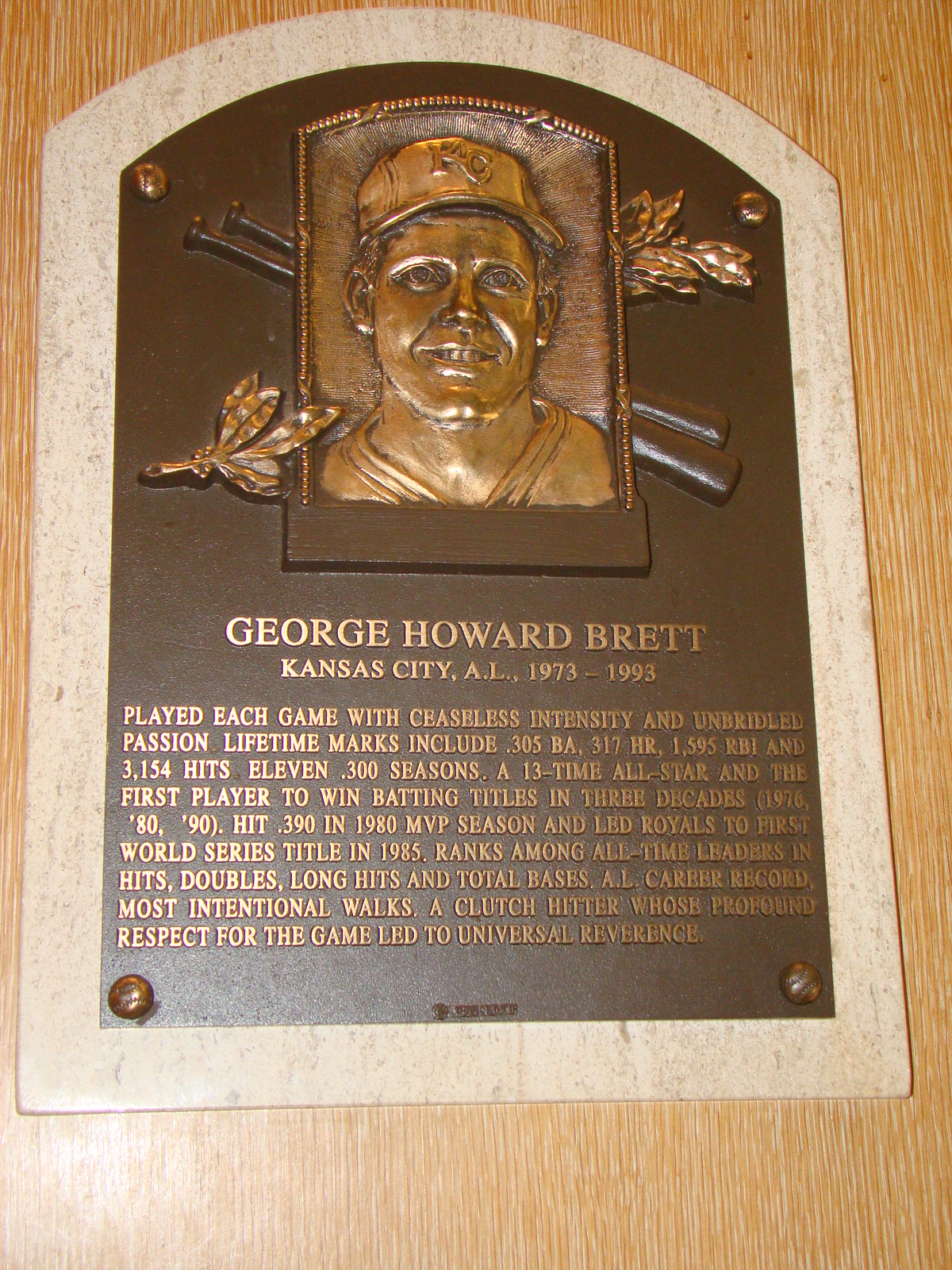This image features a detailed copper plaque mounted on a light, vertically-striated wooden background. The plaque itself has a tan outer frame and a dark brown center, with most inscriptions and the central image in a golden hue. The focal point of the plaque is a 3D embossed headshot of George Howard Brett, prominently wearing a baseball cap marked with the letters "KC," indicating his affiliation with the Kansas City Royals. Behind him, two bronze baseball bats are crossed in an 'X' shape, accompanied by gold greenery that adds to the decorative element. Below the image, text details Brett's illustrious career, stating:

"George Howard Brett, Kansas City AL, 1973 to 1993. Played each game with ceaseless intensity and unbridled passion. His lifetime marks include leading the Royals to their first World Series title in 1985. He ranks among all-time leaders in hits, doubles, extra-base hits, and total bases, and holds the AL career record for most intentional walks. A clutch hitter whose profound respect for the game led to universal reverence."

The plaque is secured to the wooden panel by four bolts and features both a detailed summary of Brett's achievements and homage to his enduring legacy in baseball.